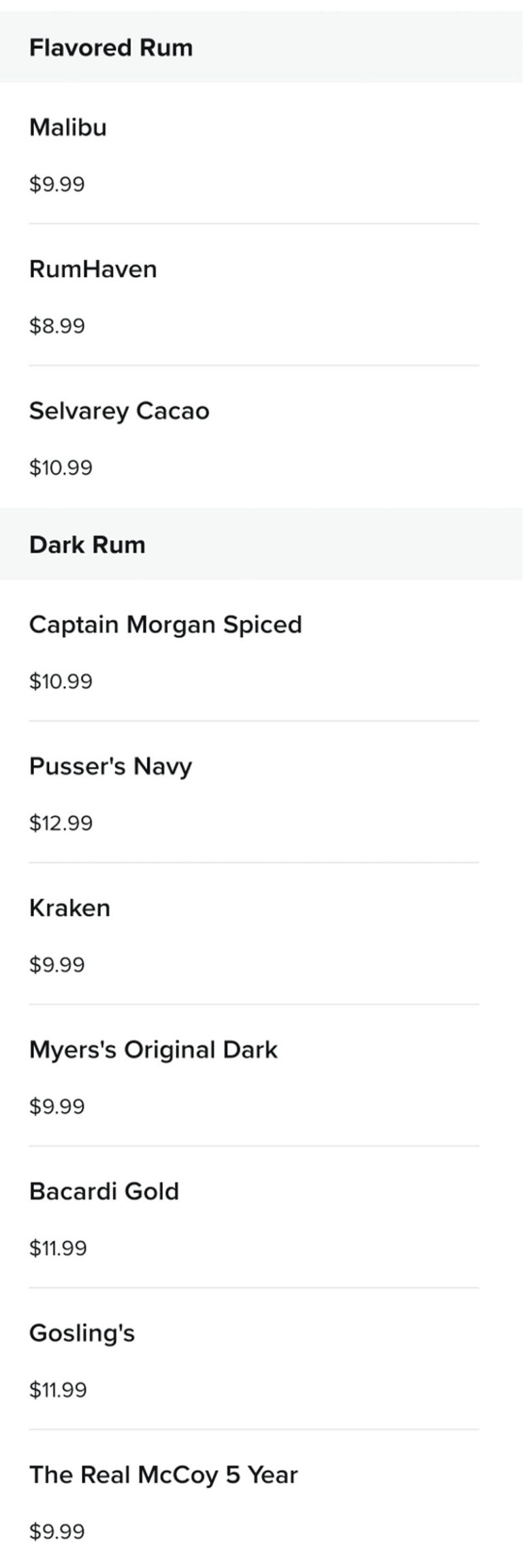The drink menu is presented with organized simplicity, set against a stark white background with all text in black. The menu header, "Flavor Drum," stands out on a very light gray background. Below this, the menu lists a variety of drinks with specified prices, each separated by very thin, light gray lines:

- **Malibu** - $9.99
- **Rum Haven** - $8.99
- **Silvery Cacao** - $10.99

A medium gray bar breaks the listing, featuring "Dark Run" in black text.

- **Captain Morgan Spiced** - $10.99
- **Pusser's Navy** - $12.99
- **Kraken** - $9.99
- **Meyers Original Dark** - $9.99
- **Bacardi Gold** - $11.99
- **Gosling's** - $11.99
- **The Real McCoy Five Year** - $9.99

The meticulous layout and minimalistic design emphasize clarity and readability, ensuring each item and its price are distinctly visible.